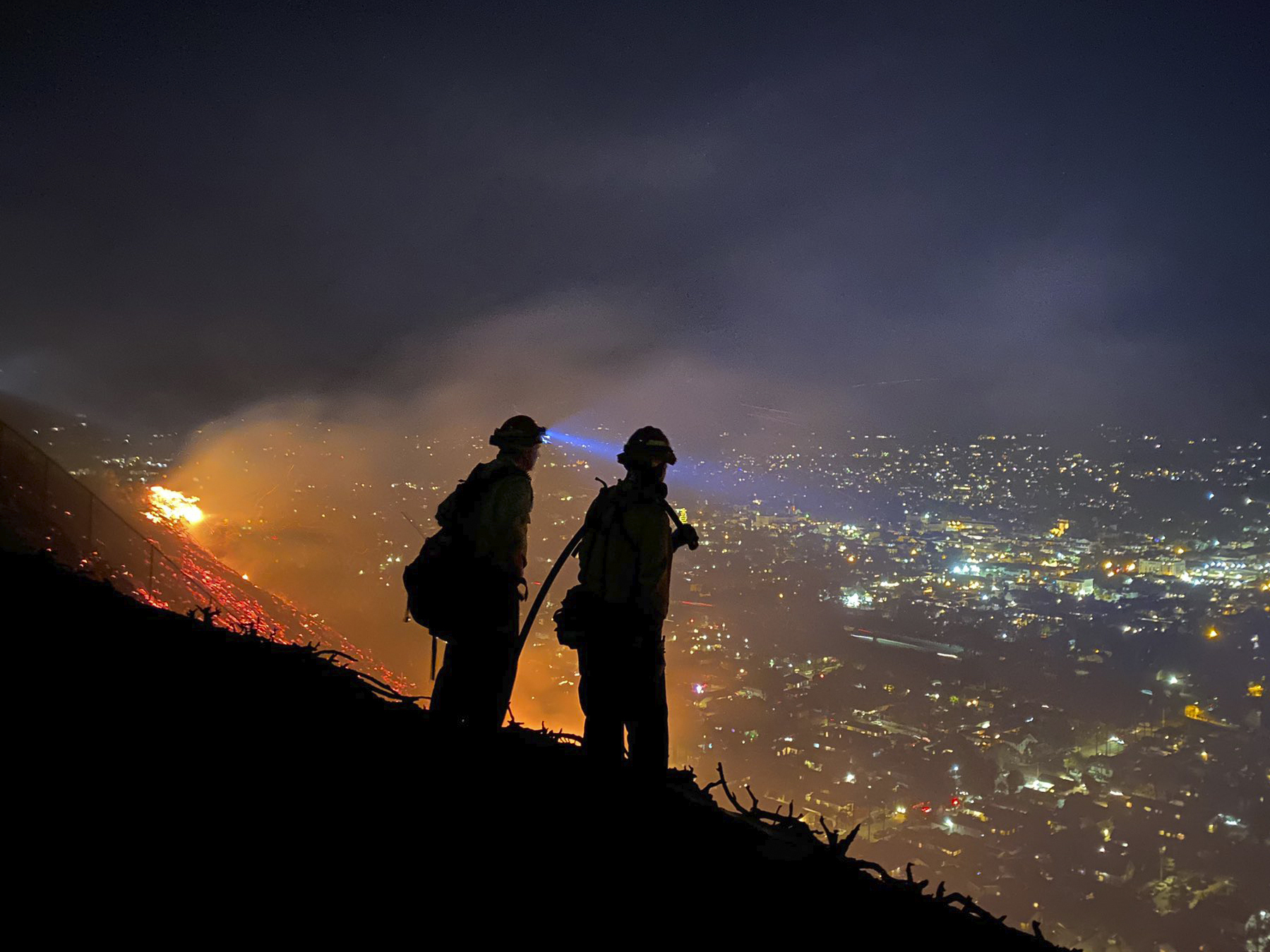A nighttime photograph captures a dramatic scene of two firefighters silhouetted on a mountainside, gazing out over a well-lit cityscape that may be Los Angeles. The firefighters, enshrouded in shadows, stand prominently in the center foreground. To their left, a raging fire emits bright white and orange flames, with billowing smoke drifting to the right, partially obscuring the city lights below. The hillside where the firefighters stand is cloaked in darkness, creating a stark contrast against the illuminated night sky and the fiery embers glowing beneath the flames. A vibrant blue light, possibly from one of the firefighter's helmets, adds a striking accent to the scene. The image artfully juxtaposes the serene, twinkling cityscape with the perilous, destructive force of the fire, highlighting the bravery and plight of the firefighters as they confront the blaze.